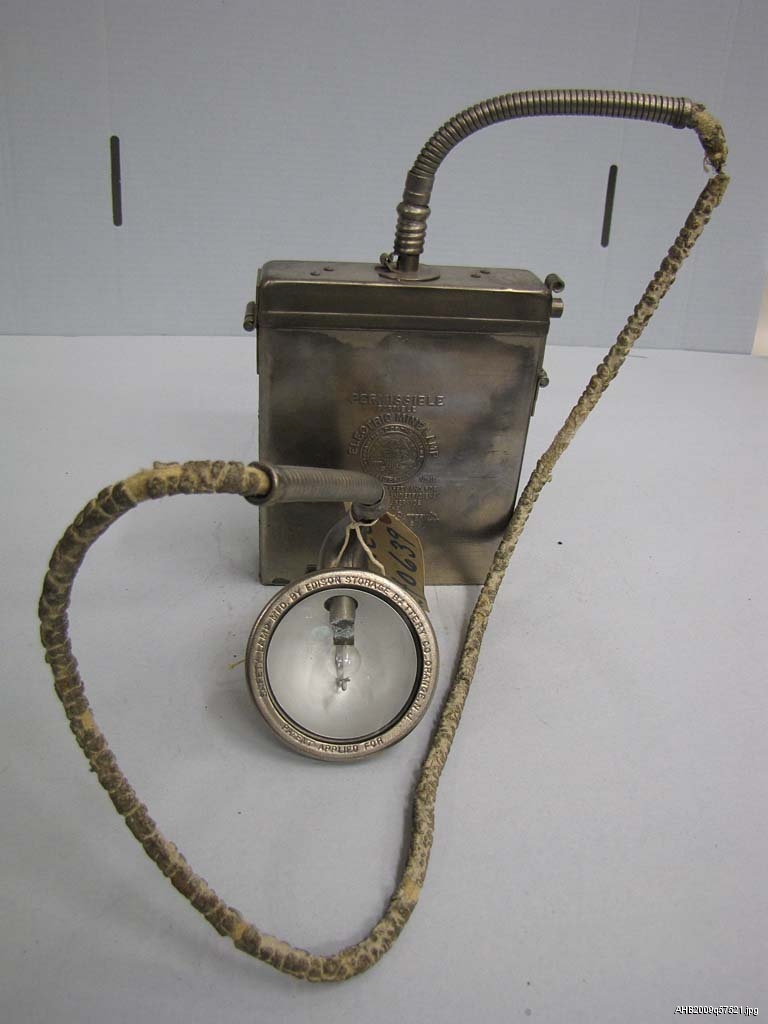The image shows a vintage, heavily worn electric mining lamp, likely on display at a museum or up for auction. The lamp features a rectangular, silver or bronze metal box with nearly illegible text that reads "Permissible Electric Mine Lamp" arranged in a circular shape. The text also includes "by Edison Storage Battery Company" and "Patent Applied For," although it’s difficult to discern due to the lamp's age and wear. A damaged, fraying cable, which seems to have been made of a polymer material, connects the box to a circular light bulb encased in glass, possibly a type of old flashlight or floodlight. The background is white and the lamp rests on a white surface, set against either a white or blue backdrop, suggesting it’s being carefully documented or sold. There’s also a small tag attached to the lamp, displaying the numbers “10639” or possibly “0639,” further indicating the item’s registration, cataloging, or lot number for the display or auction.